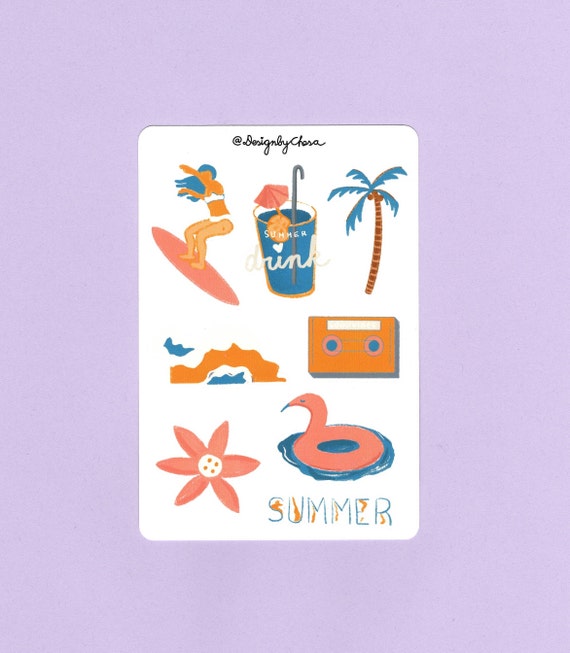The image is a vibrant, pastel-themed poster or greeting card set against a purple background. Central to the design is a white rectangular frame showcasing a lively summer scene. Inside the frame, a woman in a white bikini surfs on a pink surfboard, her skin depicted with an orange hue. To her right stands a uniquely colored blue palm tree with a brown trunk, symbolizing tropical fun. Below the tree, there is a blue drink adorned with a tiny umbrella and the label "summer drink." Adjacent to this, an orange cassette tape with blue reel dots adds a touch of vintage charm. A vivid pink flower embellishes the scene, positioned toward the bottom left.

The frame also features a variety of other summer elements, including an inflatable flamingo tube and a scenic seacoast, enriching the vacation vibe. The word "summer" appears prominently at the bottom of the rectangular frame in blue text. The imagery and typography convey a sense of joy and relaxation associated with summer activities like surfing and beach lounging. There is an Instagram handle that appears faint and reads: "design if I something," blending into the overall aesthetic. The overall design seamlessly integrates elements of summer fun, making it perfect for a seasonal greeting card or decorative poster.